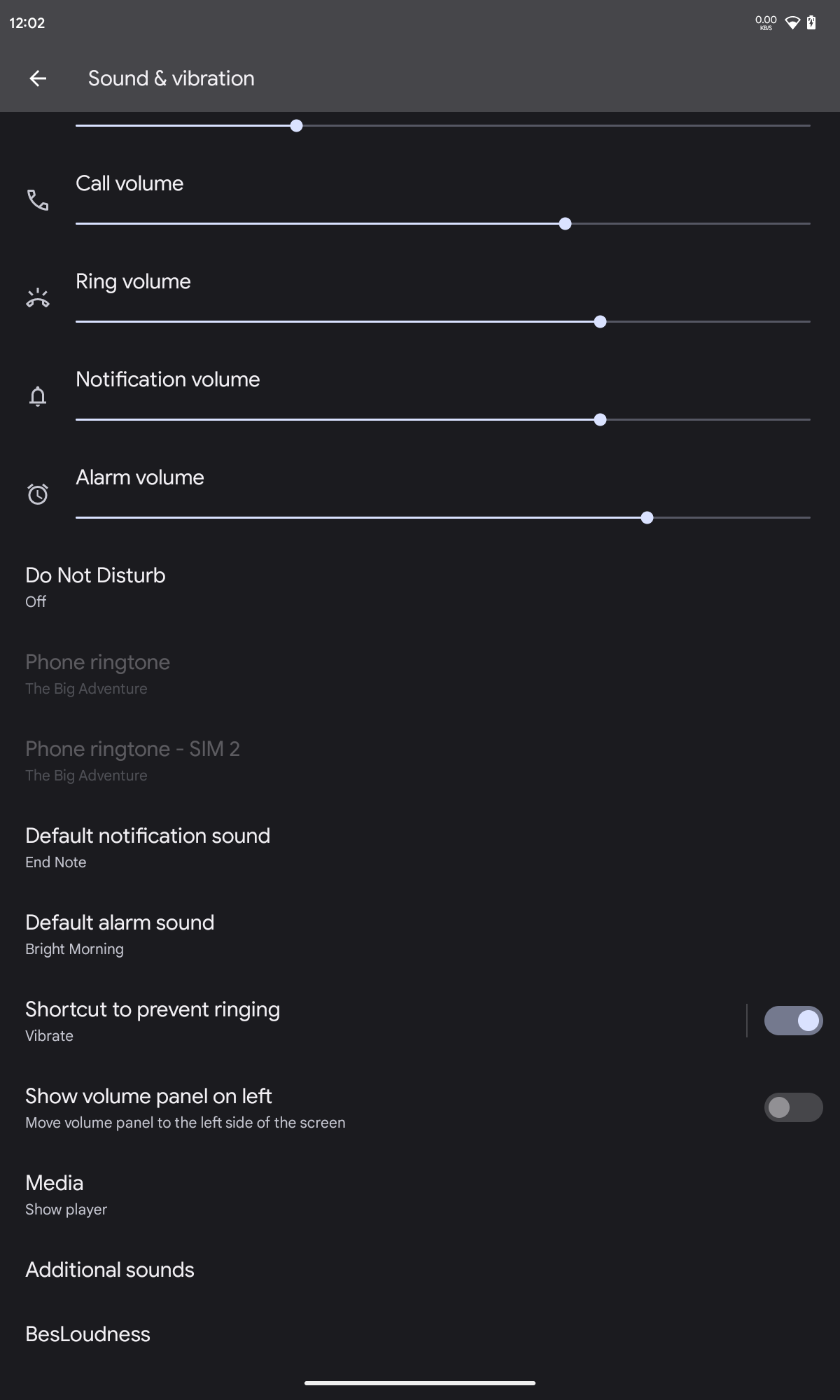The image is a screenshot of a smartphone displaying its "Sounds and Vibration" settings page. The background is predominantly black, with a dark gray horizontal rectangle at the top. The status bar at the top shows the time as 12:02, with “0.00 kevs” appearing below it, albeit small and blurry. To the right of the time, there are icons for Wi-Fi and battery status; the Wi-Fi signal is not complete and the battery level is not full either.

Below the status bar, the main content area features various volume controls represented by horizontal sliders. At the very top, an arrow pointing left is accompanied by the label "Sounds and Vibration." The sliders are used to adjust different volume settings by moving them horizontally: right for louder and left for softer. The call volume is set to about two-thirds along its line, the ring volume and notification volume match the call volume level. The alarm volume is the highest, slightly over two-thirds of the scale but not maxed out.

"Do Not Disturb" is turned off. The current ringtone for both SIM slots is "The Big Adventure," but these options are grayed out and not clickable. The default notification sound is "End Note," and the default alarm sound is "Bright Morning." The "Shortcut to prevent ringing" is toggled on, indicated by a gray elongated oval with a white dot on the right. Conversely, "Show volume panel on the left" is toggled off, shown by a darker gray oval with a gray dot on the left.

The bottom of the screen lists additional options, such as "Media," "Show Player," "Additional Sounds," and "Best Loudness" (written as a single word). No further text is present on the screen.